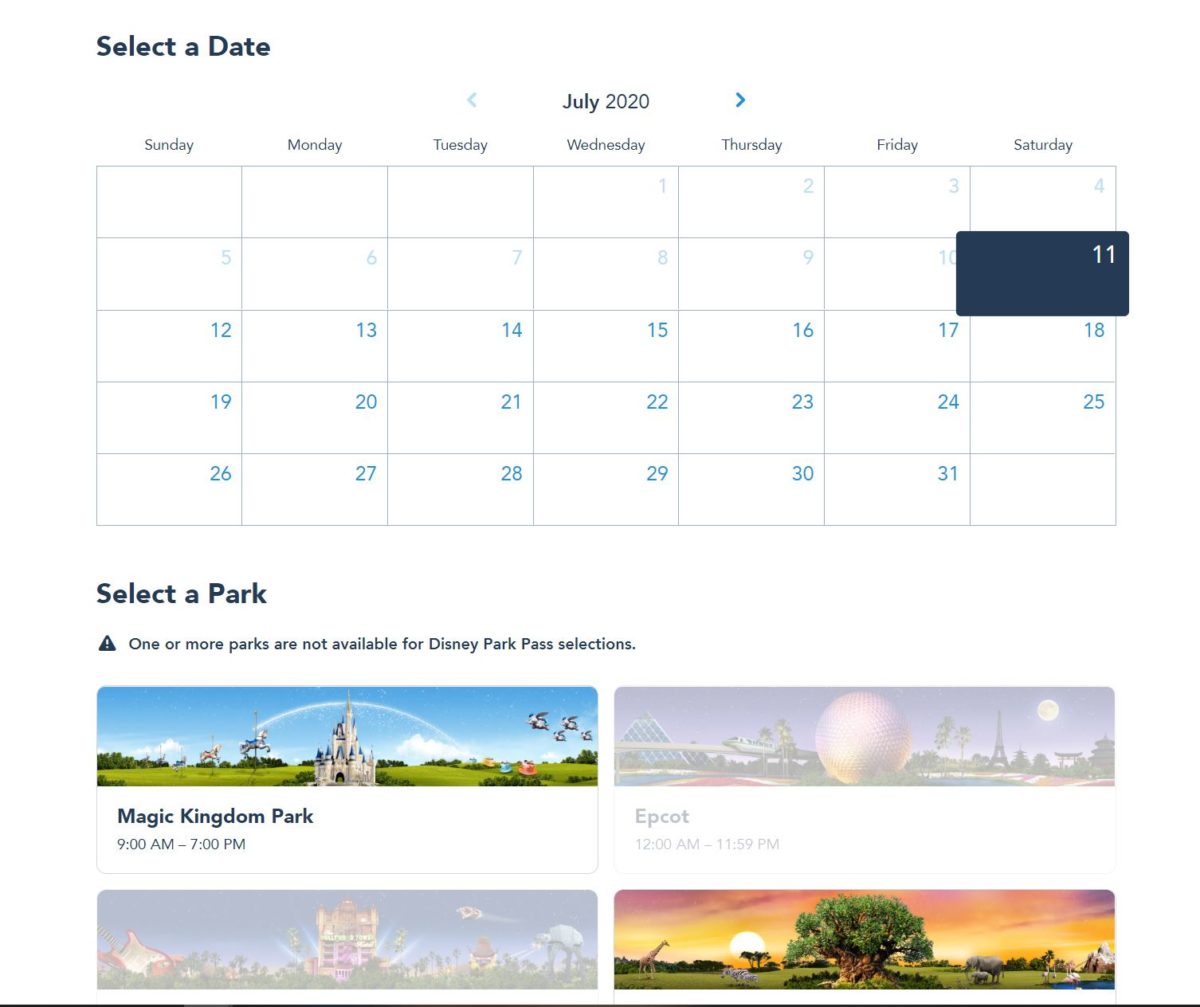The image depicts a calendar for July 2020. At the top left, a selected date is highlighted in a very dark blue or black. The month "July 2020" is centered below this section, flanked by a left arrow and a light blue right arrow.

Below, starting from Wednesday, the days of the week—Sunday, Monday, Tuesday, Wednesday, Thursday, Friday, and Saturday—are listed. Wednesday, July 1, along with the dates through July 10, are grayed out. The 11th is emphasized with a dark blue box that appears to protrude from the image. Subsequent dates (12th to 31st) are lit up, signifying they are clickable. The 31st falls on a Friday. 

In the bottom right corner, a blank white box is visible. An adjacent message indicates that "one or more parts are not available for the Disney Park Pass selection."

Below this, four distinct boxes represent different Disney parks. The top-left box reads "Magic Kingdom Park, 9 AM to 7 PM" and features a green background with a castle with blue roofs at the center. Additional details include a yellow horse, planes, colorful peacocks, and a rainbow. 

The next box, to the right, is grayed out and signifies "Epcot, 12 AM to 11:59 PM." It showcases a large golf ball-like structure with a pyramid and the Eiffel Tower.

The bottom-left box, also grayed out, is less distinct but features shades of pink and yellow. 

The bottom-right box displays a vibrant scene with African animals against an orange and purple horizon, a thick tree with green leaves at the center, and a gray elephant to the right among other animals.